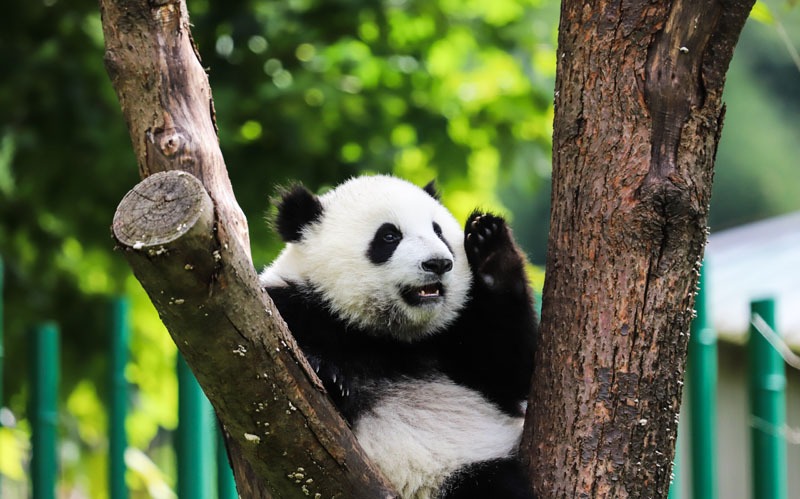This horizontal photograph captures an adorable giant panda bear sitting in the crux of a large tree, likely taken in a zoo or sanctuary. The panda, with a white face and distinctive black markings around its eyes, ears, and forelimbs, sits playfully between two V-shaped branches. The tree has a broader trunk on the right and a thick set of branches on the left, one of which has been neatly sawed off. The panda's left paw is raised, giving the impression of a friendly wave to the onlookers.

The panda appears content, its mouth slightly open, almost as if smiling and showing its lower teeth. The blurred background highlights green trees dappled with bright sunlight and green vertical bars, which likely form part of the enclosure. The setting indicates a well-structured exhibit without visible fencing, emphasizing the natural yet secure habitat for the panda. The overall composition and the panda's charming demeanor make this a very endearing photograph.